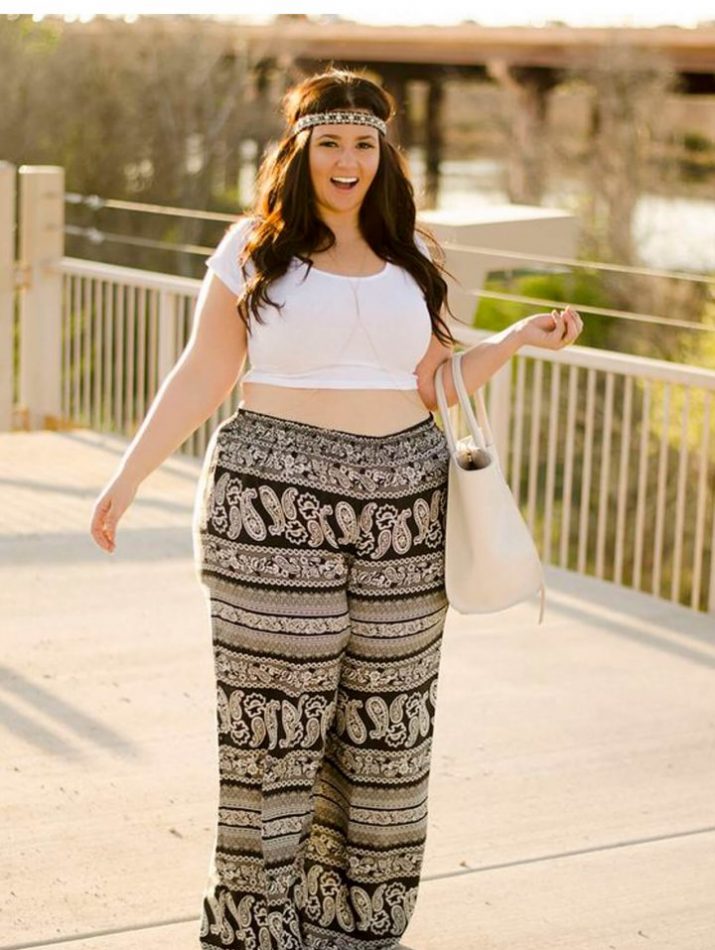In this brightly lit outdoor photograph, a woman with long brown hair stands on a cement deck under a sunny sky. She faces the camera with a cheerful smile and appears to be speaking. Her outfit is distinctive and stylish: she wears a white, tight-fitting tank top paired with loose, black-and-white patterned pants. These pants feature horizontal stripes with intricate, almost oriental-style designs. Her coordinated look is completed with a black and white decorative headband that matches her pants, and she carries a large white handbag on her arm.

The deck, where she stands, has white metal railings with two safety wires running along the top and tan posts holding them up. In the background of the image, a highway overpass stretches from left to right, and the surroundings include trees, possibly some water, and additional roads, giving the impression of being on or near a bridge. The overall scene is filled with warmth and vibrancy, capturing a moment of carefree happiness.